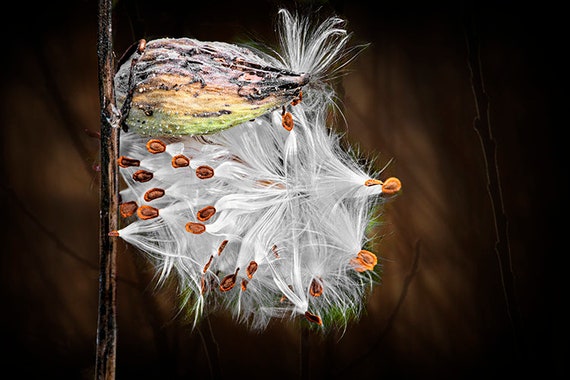The image captures a close-up view of a milkweed pod prominently positioned to the left of center against a dark brown backdrop. The pod, a defining feature of the plant, has opened to reveal a fluffy white interior that holds numerous tiny, flat seeds, colored in shades of brown and rust. The seed pod itself exhibits multiple hues, including black, green, and orange, and appears weathered, likely dried up for the fall season. The delicate, cotton-like substances emanating from the pod indicate it has already bloomed. Additionally, a slender twig, which the pod is connected to, extends from the lower part of the image, while the background remains simple and uncluttered, emphasizing the intricate details of the pod and its contents.